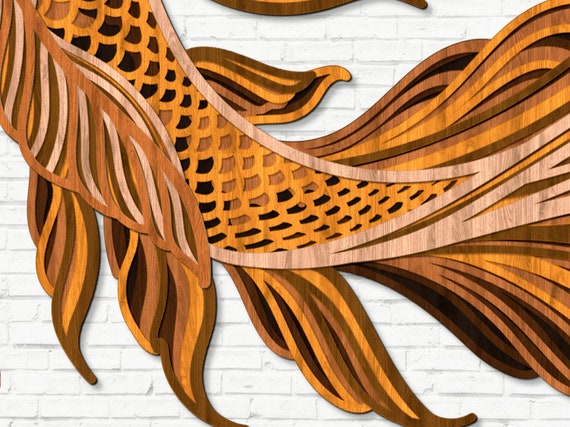This image depicts a sophisticated and elegant wooden sculpture mounted on a freshly painted white brick wall. The artwork, which intricately resembles the tail fin of a fish or perhaps a mermaid, commands attention with its gracefully flowing form. Its design includes detailed scales and swirly fin extensions, creating a dynamic sense of movement and texture. Varying hues of brown—ranging from tan and dark brown to a subtle orangey brown—contrast strikingly with the stark white backdrop, enhancing the overall visual appeal. There are also hints of black and possibly a touch of pink, adding layers to the color palette. The fin sweeps from the bottom right to the upper left of the frame, capturing the viewer's eye with its elegant, swooshy details. The honeycomb hive pattern adorning the body adds depth and intricacy to the piece, making it a tasteful and captivating work of art.